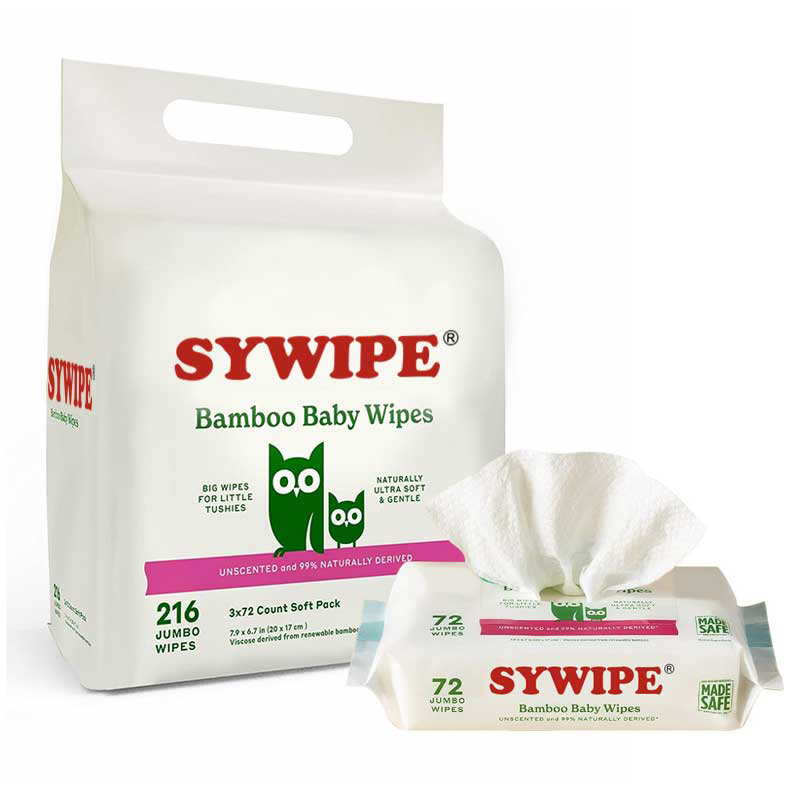This high-quality studio image, set against a pristine white background, is an advertisement for SYWIPE Bamboo Baby Wipes. On the left, there's a large, squared-off white bag with an oval handle at the top. The bag features the brand name "SYWIPE" in red font, with a trademark symbol next to it. Beneath it, the text reads "Bamboo Baby Wipes," followed by the phrases "Big Wipes for Little Tushies" and "Naturally Ultra Soft and Gentle." Centered on the bag, a green owl parent and child icon sit on a pink log, with the words "Unscented and 99% Naturally Derived" in white font on the log. Additionally, the packaging indicates it contains 216 Jumbo Wipes, divided into three packs of 72 wipes each. To the right of the large bag is a smaller, rectangular pouch from which a single wipe is artistically pulled out in a fan-like shape. The packaging predominantly features green, red, white, and pink colors, enhancing the clean and gentle aesthetic of the baby wipes product.